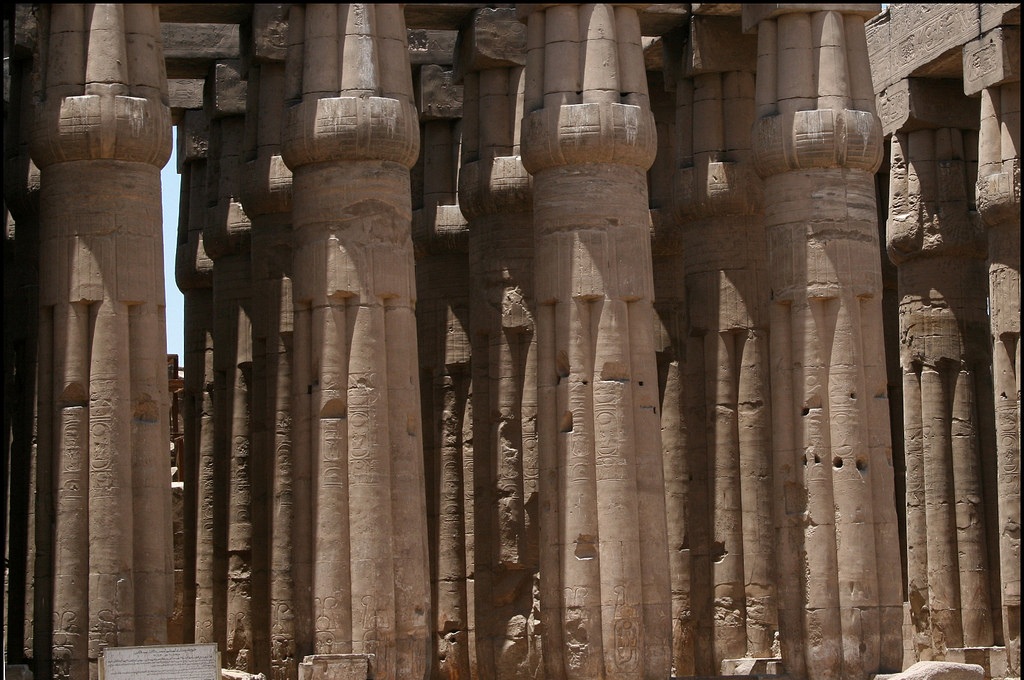This photo, taken in Egypt, focuses on a close-up view of the ancient pillars at Luxor Temple. The image prominently features four massive limestone columns in the foreground, each intricately detailed with vertical lines that give them a scalloped appearance. The columns expand upwards with rings and rounded sections, showcasing their uniform shape and size. Behind this front row, three more similar columns can be seen, creating a pattern that extends into the background. Additionally, horizontal beams stretch across the tops of these columns, indicating structural connections.

The setup appears to be part of an outdoor display, with a small, blurry sign featuring black text on a white background situated at the bottom left corner of the photo. The columns, composed of smaller segments, bear ancient carvings and designs, including drawings and symbols. Many columns exhibit signs of aging, with visible chips and worn areas, particularly at their bases. Further to the right side of the image, more columns are visible, arranged in several rows that recede into the background. The overall scene is bathed in natural light, with glimpses of a blue sky peeking through the spaces between the columns, lending a timeless and venerable atmosphere to the temple remains.